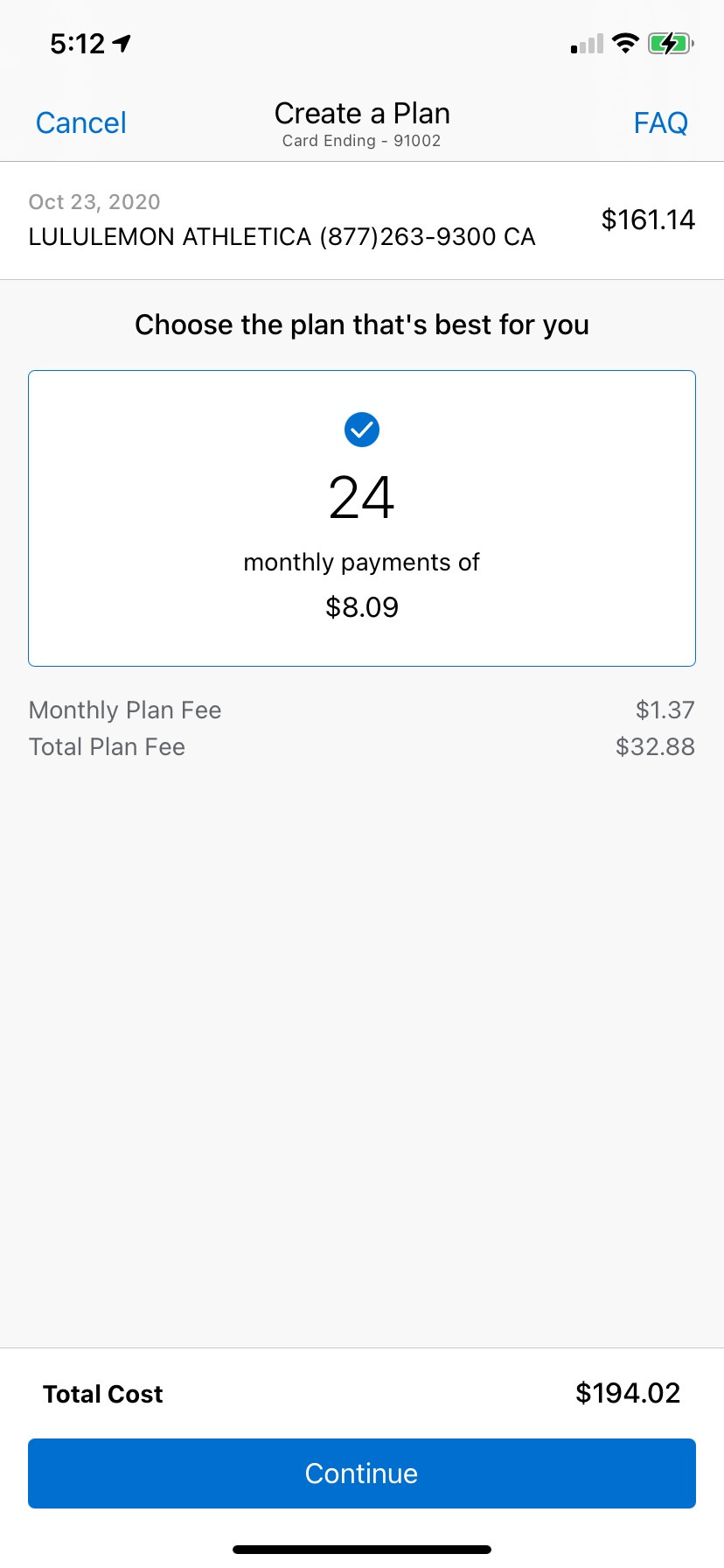The image features a green screen with a gray background displaying detailed information about a subscription plan. Prominent elements include a battery icon showing that the battery is charging, indicated by a thunder symbol and marked 512. 

At the top, the image references an event on October 23rd, 2020, linked to Lululemon Athletica. A phone number, (877) 263-9300, is also displayed.

Below, the main section is dedicated to subscription plan options:
- "Choose the plan that's best for you" is highlighted within a rectangle.
- A blue circle with a checkmark symbol and the number 24 signifies the selected plan.
- Monthly payments are listed as $8.09.
- Additional monthly plan fees are $1.37.
- The total plan fee sums up to $32.88.
- The total cost of the plan is calculated to be $194.02.

The image also features various actionable options in blue text, including "Cancel," "Create a plan," and "FAQ." A blue rectangle near the bottom features "Continue" in white text. Lastly, a black bar is positioned across the middle at the bottom of the image.